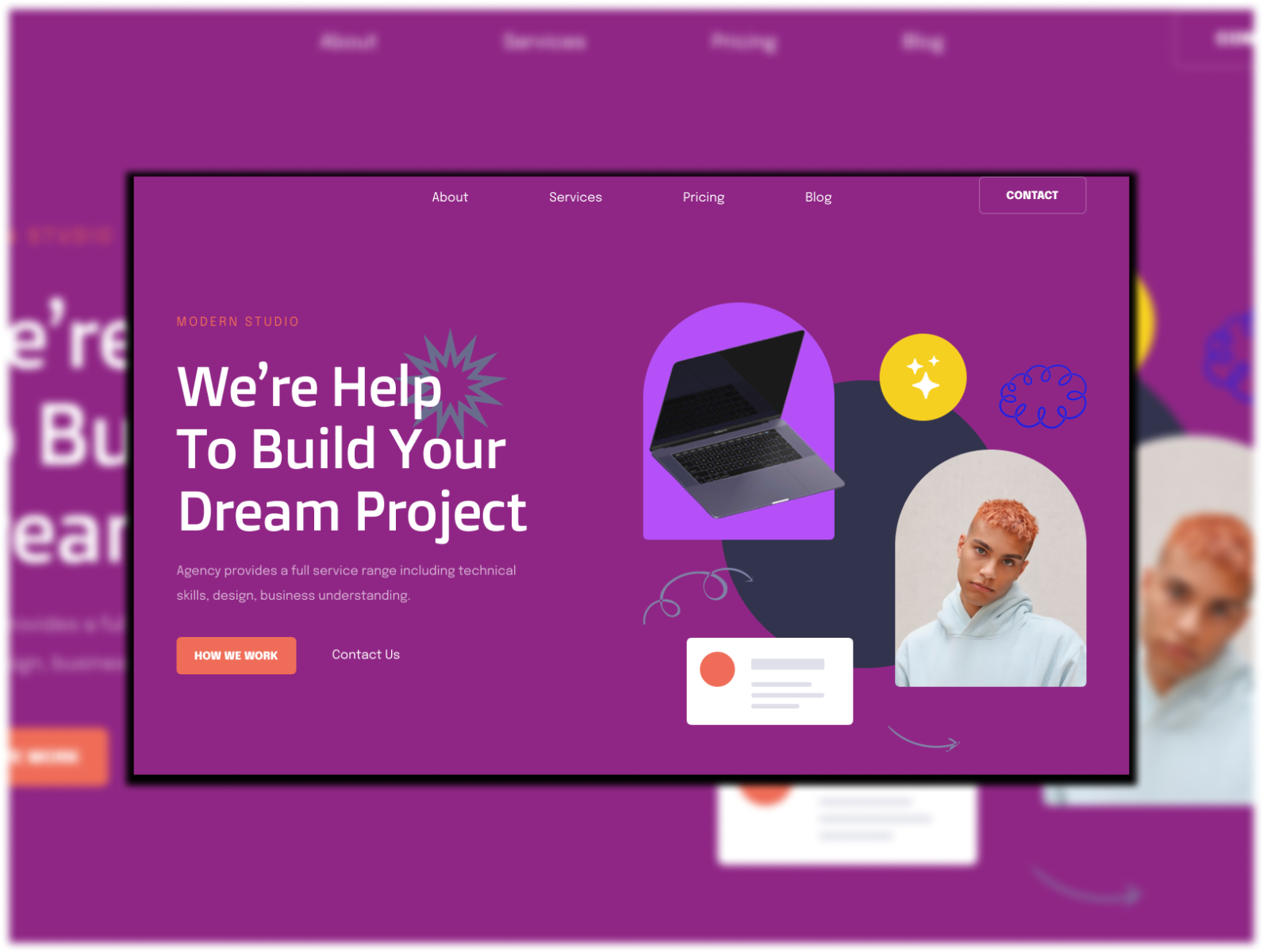The image depicts a modern studio website with a clean, professional design. The primary background is a deep purple with subtle black outer shadows that give the page depth. 

At the very top of the page, there is a navigation menu centrally aligned, featuring white text links that say "About," "Services," "Pricing," and "Blog." On the right-hand side of the navigation bar, there is a rectangular context button with a purple background.

Below the navigation menu, aligned to the left, the brand name "Modern Studio" is displayed prominently in a bold red font. Beneath this, a large white font reads, “We’re happy to build your dream project.” Adjacent to the word “Project,” a small explosion icon adds a whimsical touch.

Further down the page, there is a two-line sentence that appears to describe the agency's offerings, though it's partially obscured. It reads, "Agency provides a full service range, including technical [unreadable text] understanding."

Directly under this text is a prominent rectangular button in orange that reads, "How we work." To its right is another call-to-action link that says, "Contact us."

The bottom section of the image includes media clips, one featuring a laptop and another of a person with short, pinkish hair, turned slightly to the side, wearing a white hoodie.

The overall design is sleek and modern, with a consistent purple color palette accented by red and orange highlights for important interactive elements.